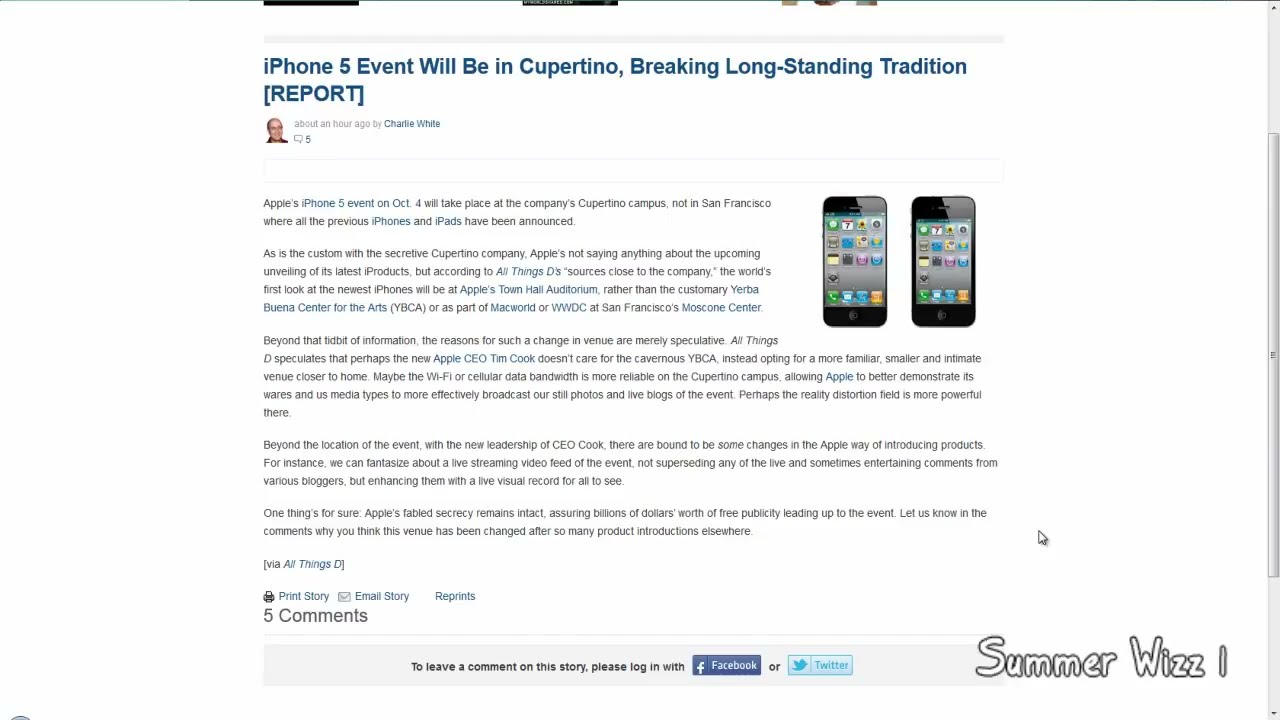This image is a screenshot of a computer screen displaying a web page with a completely white background. On the right side, there is a thin gray scroll bar. The image's top edge is cut off slightly. Prominently in blue text in the top middle of the screen, the headline reads, "iPhone 5 event will be in Cupertino, breaking longstanding tradition. Report." Below this headline is a smaller gray text indicating "about an hour ago by" followed by the blue text "Charlie White." Adjacent to this, on the left, is a small picture of a man's head, likely the author, Charlie White. To the right and slightly downward, there are images of two iPhones side by side—one appearing slightly larger than the other, with their screens displaying various apps. To the left of these images, the article is composed of five paragraphs detailing the event. At the very bottom of the screen, it is indicated that five comments have been left on the article, and there are social media links for readers to log in with Facebook or Twitter to leave their comments. Additionally, in the lower right-hand corner, the text "summer whiz one" can be seen, possibly indicating the name of the website or section.